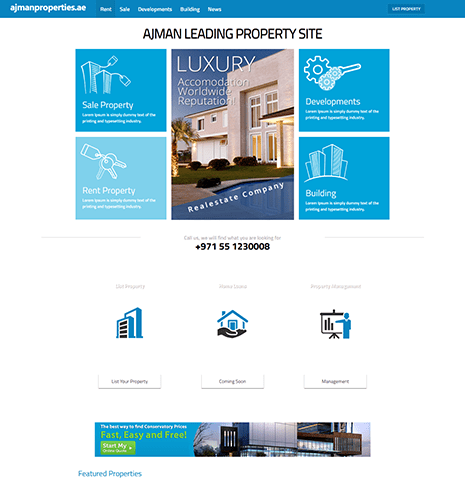**Detailed Caption:**

This image is a screenshot of the Ajman Properties website. The title of the site, "ajmanproperties.ae," is displayed prominently at the top left corner. The website features a horizontal blue menu bar with several navigation buttons. Although slightly blurred, the first button reads "Rent" and is darkened, indicating the active section of the website. Other buttons likely include "Sale," "Developments," "Building," and "News." On the far right, there's a dark blue button with some reference to properties.

Beneath the menu bar, centered on the page, the name of the website or company is displayed as "Ajman Leading Property Site." Below this header, there is a visually-structured section featuring five images:

- On the left, two vertically stacked images: 
  - The top image, in dark blue, labeled "Sale Property," depicts two buildings with price tags.
  - The bottom image, in light blue, labeled "Rent Property," shows a set of keys.

- The central image showcases a modern-style house with a green lawn and a snippet of what seems to be a pool. The caption reads "Luxury Accommodation Worldwide Reputation," with a subtitle "Real Estate Company."

- On the right, two additional vertically stacked images:
  - The top image, shaded in blue, shows ranches and labels the "Developments" section.
  - The bottom image, depicting cartoon buildings, represents the "Building" section.

Below these images, a contact phone number is provided, alongside three icons for additional options:
- A building,
- A hand holding a house,
- A person observing a chart.

Each icon seems to link to different informational sections, although the text is blurry. At the bottom of the page, an advertisement bar promises that browsing prices on the website is "fast, easy, and free."